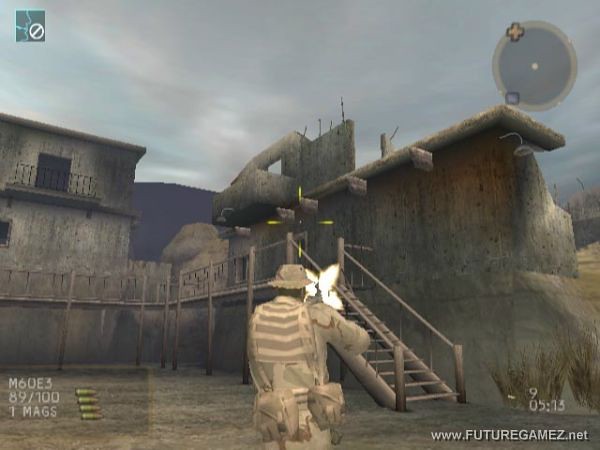The image depicts a scene from a video game where a player character in brown military gear, including a tan fedora and utility belt with various bags and casings, is firing a gun that produces tracer rounds and visible flames. The character stands on gray ground in front of a wooden staircase that ascends to a ledge connected to a structure resembling a jail building. The environment consists of rundown, beige-gray buildings under a cloudy, gray sky. In the bottom left corner of the screen, "M60E3" is displayed above "989/100" and "1 mags," accompanied by four bullet icons in white text. Meanwhile, the bottom right corner features the URL "www.futuregames.net" in white. The top right corner displays a radar-like map icon with a gray circle, a white dot, and an orange cross. Additionally, there's a small square map highlighted in blue at the top left of the screen. The character appears to be aiming at the top of the structure, enhancing the immersive military-action atmosphere of the game.